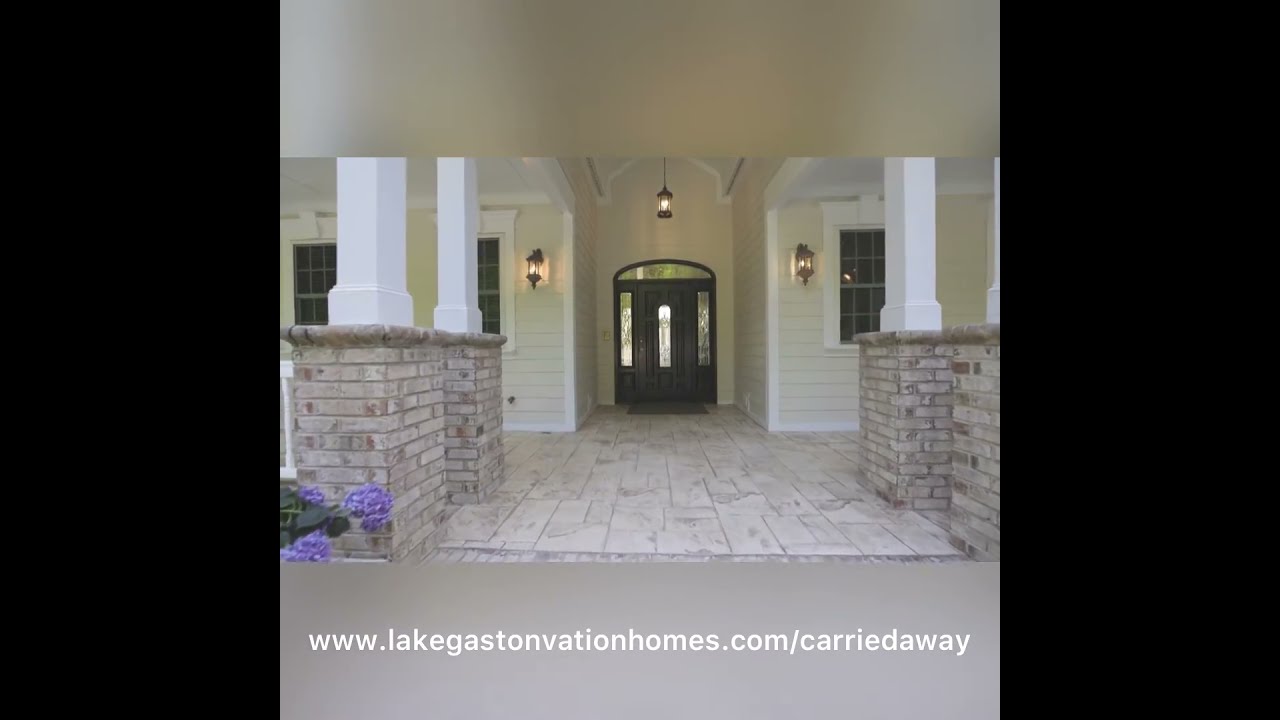The image depicts the entryway of a sophisticated and inviting vacation home, implied by the footer text "www.lakegastonvationhomes.com/carriedaway" which possibly features a typo. The focus is on the entrance, framed by large black bars on the sides and a fuzzed, grayscale header and footer highlighting the website. The home features four white columns standing on rugged red-brick bases, supporting a covered porch area. The walkway leading to the dark front door, which has four glass panels including a transom window above and two side windows, is paved with gray stone tiles transitioning from a tan concrete driveway. On either side of the front door are additional lights - three in total, enhancing the warm ambiance. A blooming purple hydrangea bush graces the bottom left corner of the image, adding a splash of color to the light gray, almost white siding of the house. A welcome mat lies before the door, completing the inviting scene.